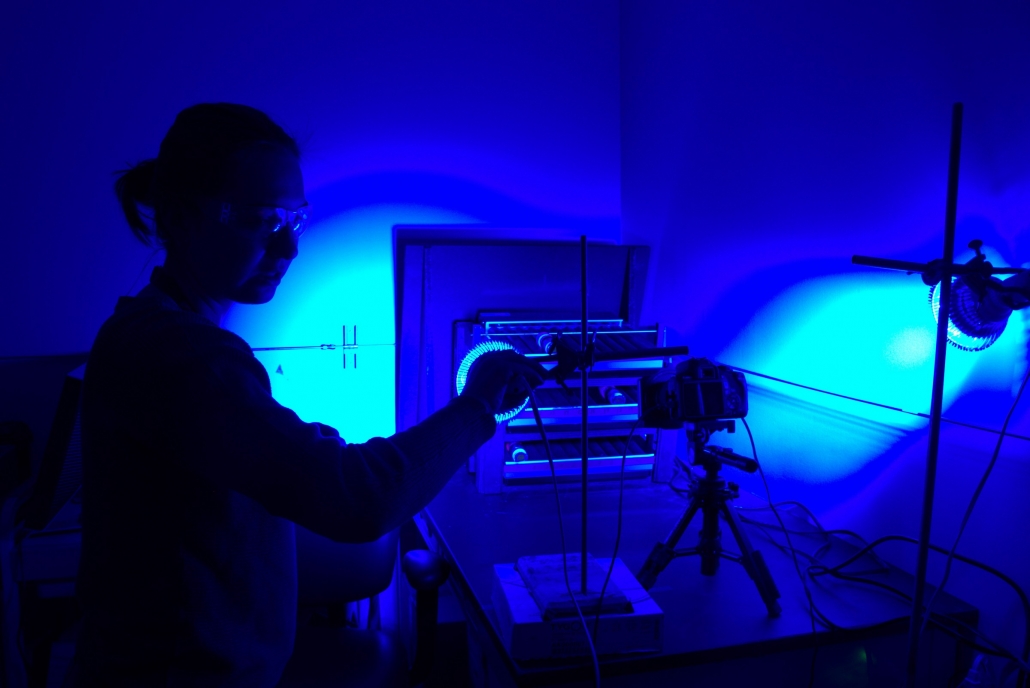This photograph depicts a dimly lit room, possibly a darkroom or a photography lab, bathed in dark violet and blue hues. In the center of the image, a person, likely a woman with her hair tied back in a ponytail, is seen from the head to the waist. She is wearing safety goggles and what might be a lab coat or a sweatshirt, though the dim lighting makes it challenging to determine. She stands on the left side of the image, her right hand raised to adjust the positioning of a leftmost spotlight. In front of her, on a large tabletop surface, there are two spotlights casting a soft sky-blue light on the back wall. Nestled between these spotlights is a camera mounted on a tripod, aiming at three stacked metal trays at the back of the table. The overall setting suggests a careful arrangement, likely for photographic documentation or experimentation.